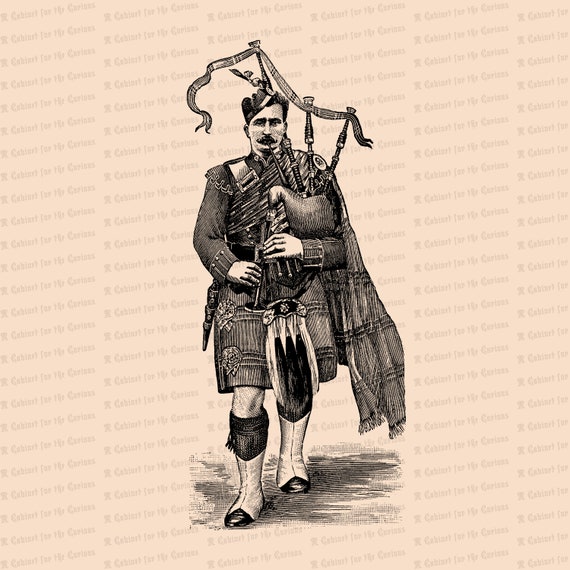This is a finely detailed black and white drawing on a cream-colored background, depicting a man marching toward the viewer while playing the bagpipes. He is dressed in full Scottish regalia, including a short, striped kilt, a long-sleeved jacket adorned with various buckles and shackles, and a cape hanging off his left shoulder. His attire suggests he could be part of a military procession or parade. He wears a hat tilted sideways on his head, and his facial features include short dark hair and a dark mustache. The bagpipes he is playing are intricately detailed, with a ribbon connecting the three pipes that extend over his shoulder. His black and white shoes have black toes facing forward. The man’s hands are positioned at his waist, and he is actively blowing into the bagpipe’s mouthpiece. Shadows are skillfully sketched at the bottom to give a sense of ground. Though there are faint rows of black lettering in the background and a watermark, the text is illegible.